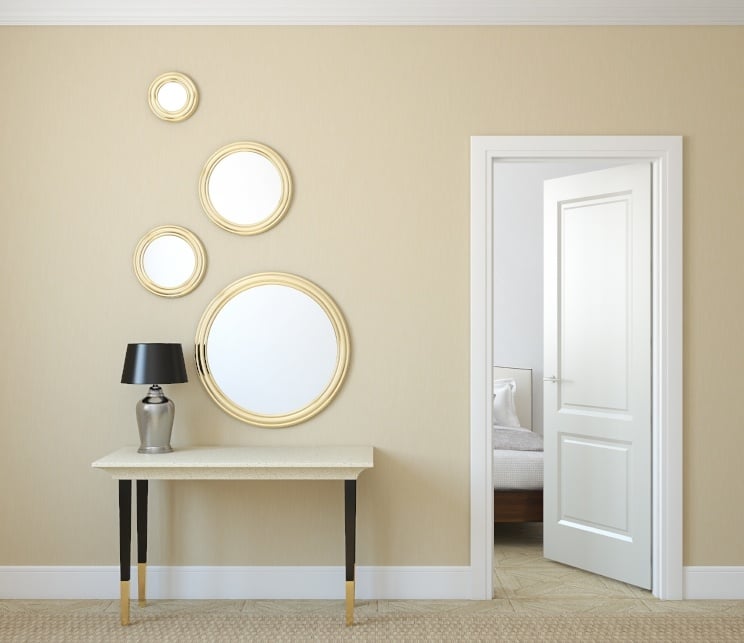The photograph showcases the modern, neutral-toned interior of a home, capturing what appears to be the hallway outside a bedroom. The walls are adorned with taupe wallpaper, and a cream-colored wall features four round mirrors of varying sizes, arranged decoratively like bubbles with gold frames. Below the largest mirror is a stylish white hallway table with distinctive black legs that transition to a natural wood finish at the very bottom. On the left side of the table sits a small stainless steel lamp with a dark gunmetal metallic shade. The hallway is carpeted in light brown, while the visible bedroom beyond an open door on the right has a tiled floor and lacks carpeting. The baseboards line the walls, adding to the room's refined decor. The view through the door offers a glimpse of a bed, hinting at the connected bedroom.